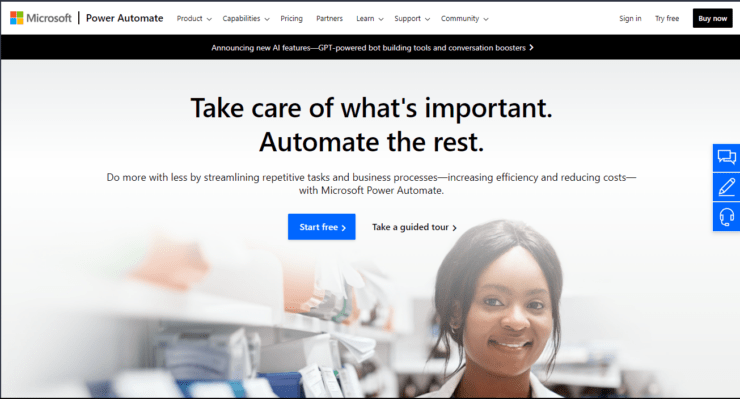The homepage of the Microsoft Power Automate website has a sleek, professional design featuring a black banner at the top. The banner announces new AI features, specifically highlighting GPT-powered bot-building tools and conversion boosters. Below the banner, the main image prominently displays an African American woman against the backdrop of shelves, conveying a sense of productivity and efficiency.

The tagline next to her image reads, "Take care of what's important. Automate the rest. Do more with less by streamlining repetitive tasks and business processes, increase efficiency and reduce costs." This succinctly captures the essence of what Microsoft Power Automate aims to offer its users.

The navigation bar at the top of the page includes a variety of options: Product, Capabilities, Pricing, Partners, Learn, Support, Community, Sign in, Try for Free, and Buy Now. These are organized as pull-down menus, offering a comprehensive overview of what the service entails.

A prominent blue button labeled "Start here" invites users to initiate their journey with Power Automate. Next to it, a black button labeled "Take a guided tour" offers an introductory walkthrough.

To the right, a set of three blue buttons depict icons for different communication options: one with a speech bubble for chat or text, one with a pencil likely for drafting messages or notes, and one with headphones indicating customer service support. These could represent functionalities related to chatbots, email, and phone support.

The color palette of the website utilizes a range of hues including blue, black, yellow, red, green, gray, and white, creating a visually appealing and professional layout.